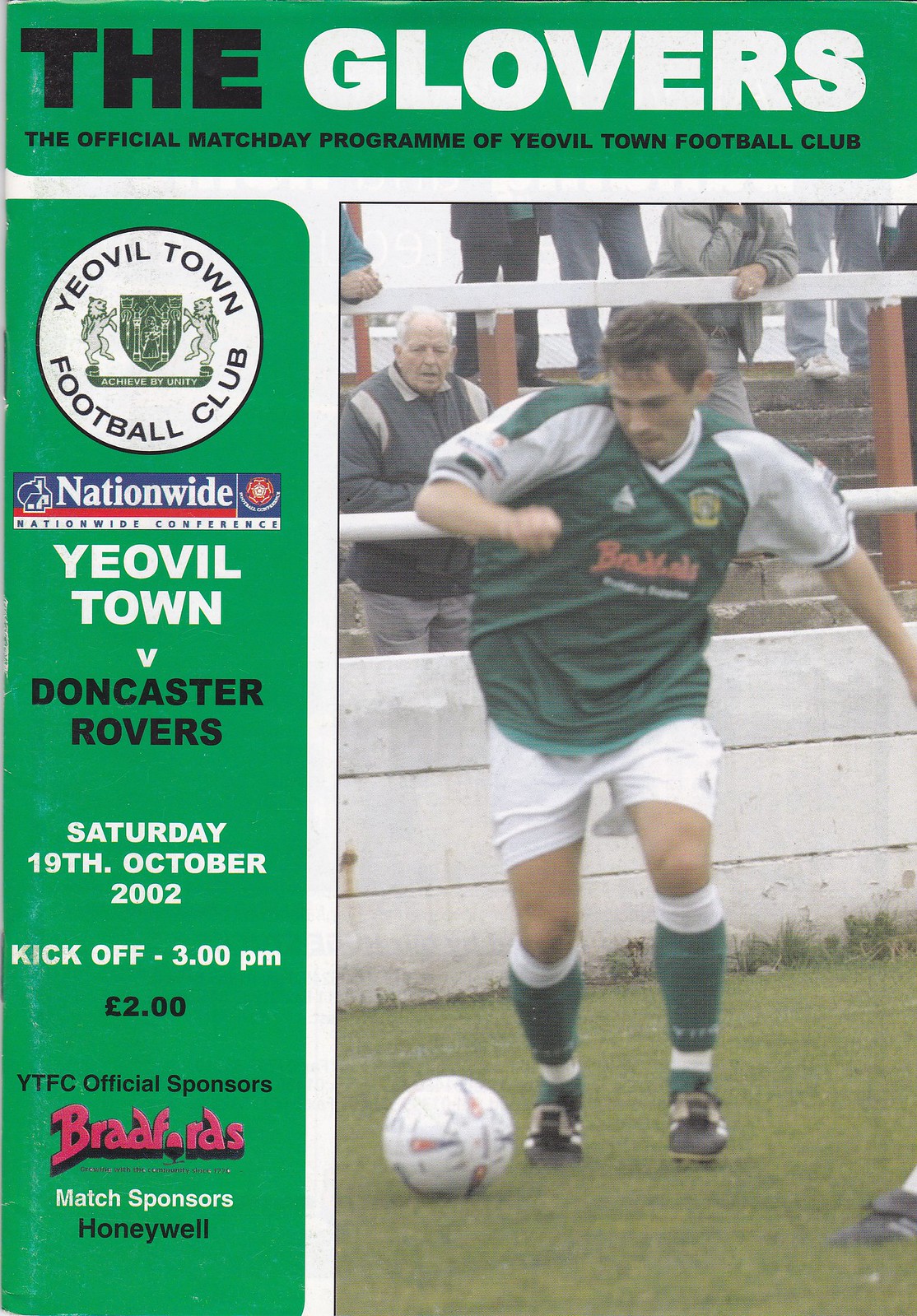The poster predominantly features a green background, highlighting its theme centered around the Yeovil Town Football Club. The header at the top of the poster reads "The Glovers," with "The" in black and "Glovers" in white. Directly beneath this, in a smaller black font, it reads "The official match day program of Yeovil Town Football Club." The word "Yeovil" is spelled out as "Y-E-O-V-I-L."

On the left side of the poster, there is a green vertical section containing the Yeovil Town Football Club logo, which is a white circle outlined in black with the club's name inside. This section also includes the Nationwide conference logo, an advertisement. Below this, it details the match: "Yeovil Town v. Doncaster Rovers, Saturday 19th October 2002, kickoff 3pm," along with a mention of the official sponsors.

The right side of the poster features an action photograph of a white male soccer player with brown hair. He is dressed in a green-and-white short-sleeved jersey, white shorts, green knee-high socks, and cleats, appearing ready to kick a soccer ball. In the background, spectators can be seen in the stands, adding to the lively atmosphere of the scene.